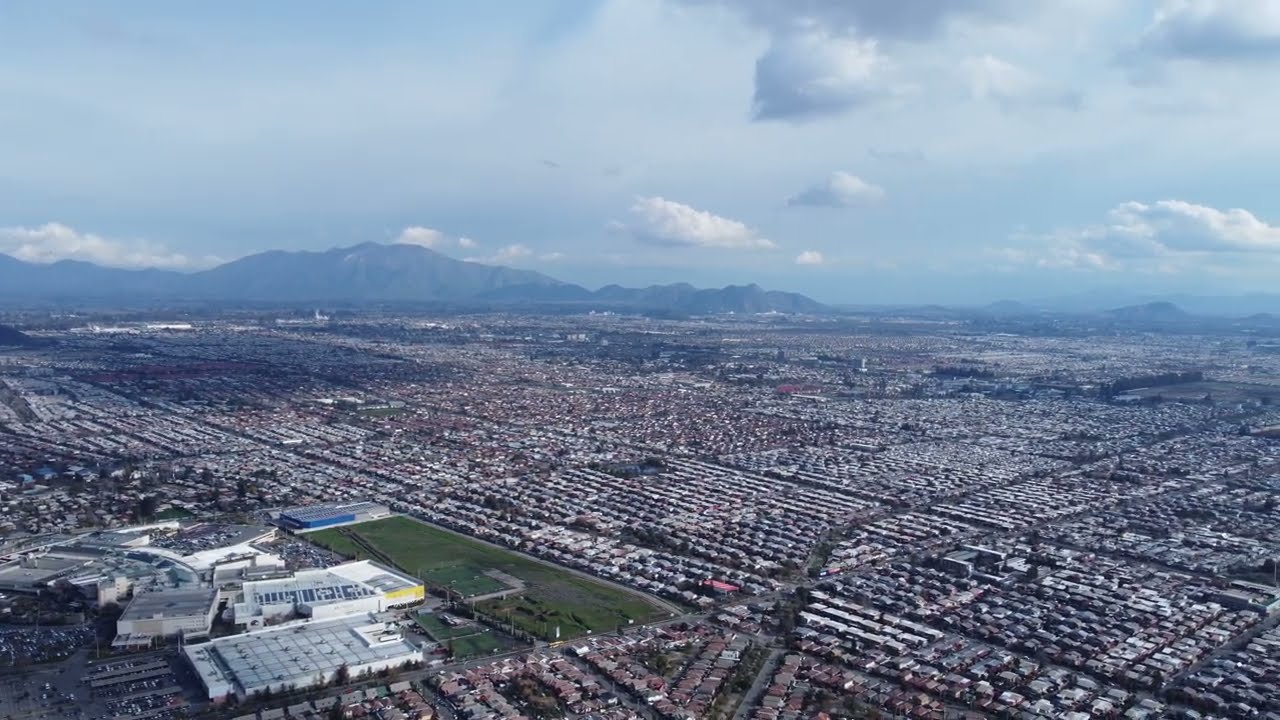This highly detailed, panoramic color photograph captures an extraordinarily congested residential area, viewed from above, likely taken by a drone. Rows of tightly packed houses stretch across the bottom half of the image, intersected sporadically by a few narrow roads, emphasizing the high population density within this urban landscape. The houses display a variety of neutral shades, including white, gray, and brown, accentuating their uniform appearance. On the bottom left corner, there is a cluster of large commercial buildings, identifiable by their light gray color and the adjacent parking deck.

A prominent feature of the scene is a significant open space in the form of a rectangular patch of green grass, possibly a playing field, situated next to a substantial structure that appears to be a school or university. This is the only notable break in the otherwise relentless sprawl of housing.

In the far distance, a dark blue mountain range stretches across the horizon, particularly evident on the left side of the image. Above, the sky is overcast with light gray tones, interspersed with darker rain clouds, especially in the upper right section. The overall photographic style is representational realism, capturing the intricate details and expansive scope of this densely inhabited cityscape.